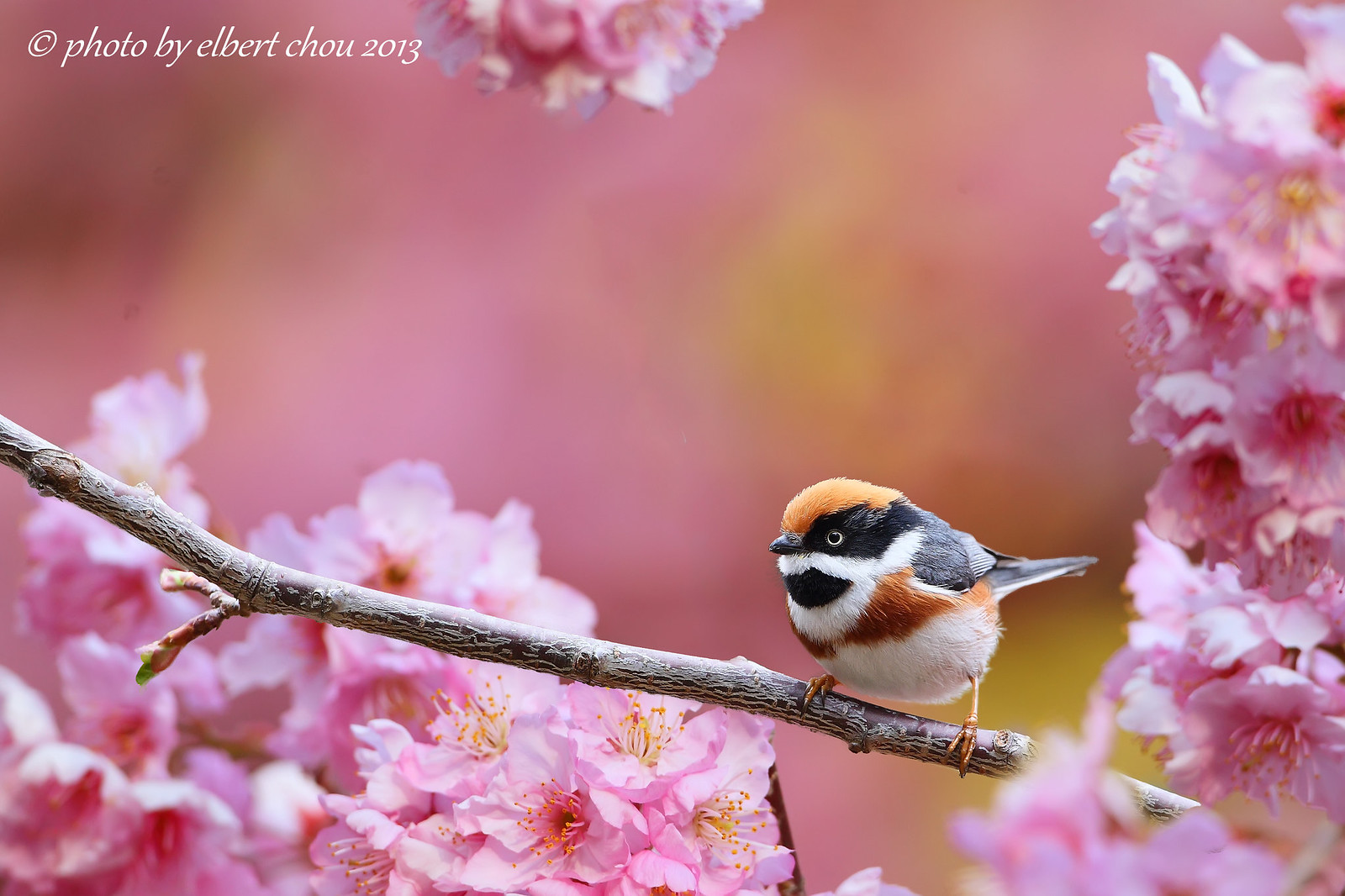This vibrant photograph showcases a small, colorful bird perched on a branch amidst an explosion of pink flowers. Dominating the scene is the rich pink hue of the background and the flowers, dotted with occasional splashes of orange. The bird, positioned slightly off-center to the right and just below the middle, features a striking mix of orange, black, and white. It has an orange head, black markings around its eyes and feathers, a white and black neck with hints of orange, and a white belly. Its tiny black bill is distinct against its intricate plumage. The branch, starting from the bottom right and extending to midway on the left, serves as the bird's perch. The blurred pink background and vibrant pink flowers envelop the bird on the left and below, with additional pink flowers hanging from the top. The scene suggests an outdoor setting, possibly a garden, on a sunny day. In the upper left corner, there is a watermark that reads, "Photo by Albert Chow, 2013."